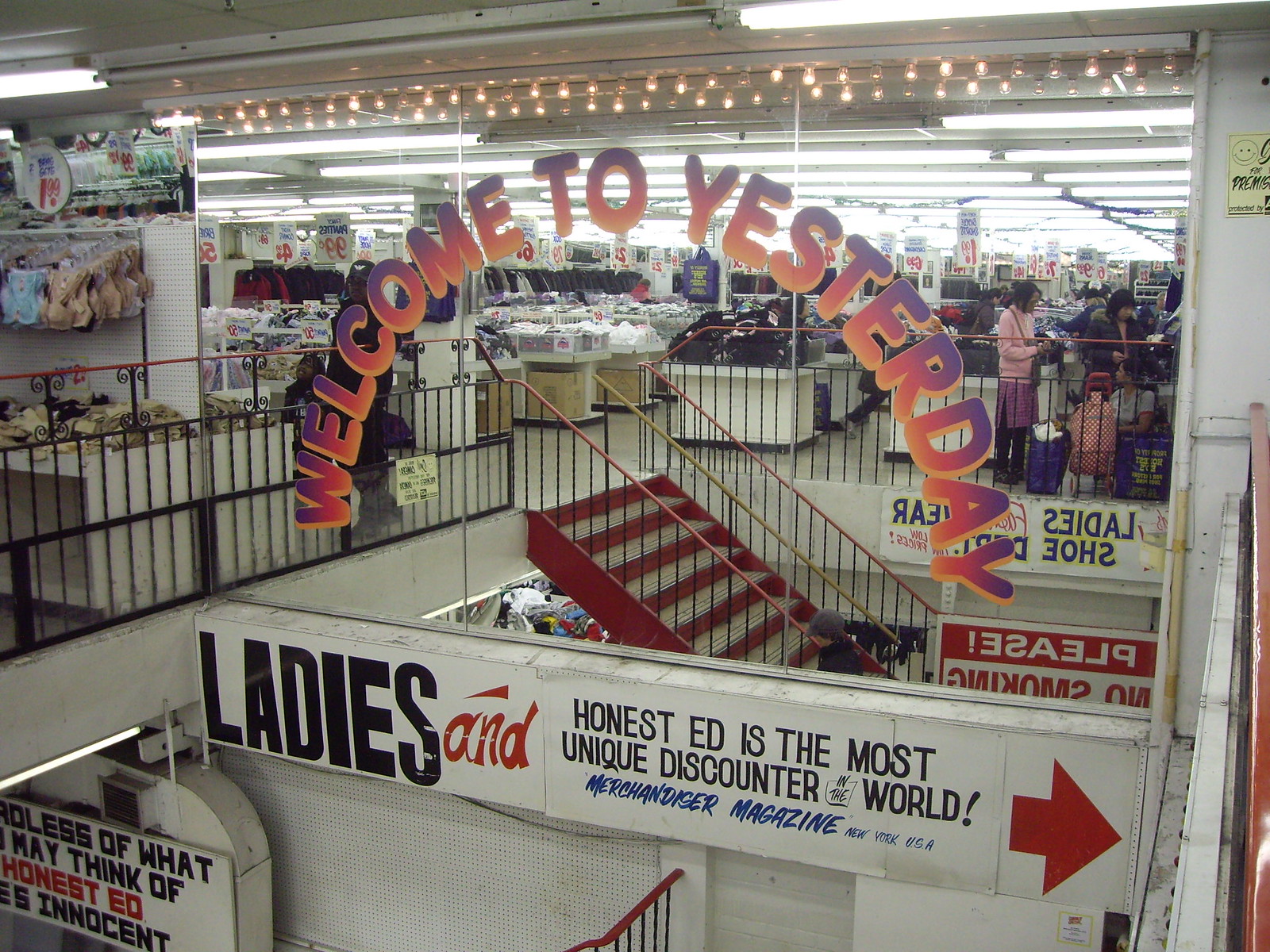This photograph showcases a store located within a bustling mall. Central to the image is the store’s large front window, emblazoned with the phrase "Welcome to Yesterday" arranged in an arch. The lettering features a gradient effect, transitioning from dark purple at the top to light pink at the bottom. Fluorescent lights illuminate the store’s interior from front to back, creating a bright and inviting atmosphere.

Below the "Welcome to Yesterday" sign, there's a soffit bearing another sign, which reads, "Ladies and Honest Ed is the most unique discounter in the world. – Merchant Magazine, New York, USA," with a red arrow pointing to the left. A partially visible sign underneath this soffit reads, "Regardless of what you may think of Honest Ed, he is innocent" alongside a "Please No Smoking" notice. Additionally, a sign for "Lady's Shoes" can be spotted, though part of it is obscured by the "Yesterday" sign.

To the right, a stairway ascends to a landing area. The stairs are flanked by a display advertising ladies' bras for $1.99, hinting at the store's affordable pricing. Inside the store, numerous racks and tables filled with various items are visible, with many products marked at 99 cents or offering significant discounts up to 50% off. The scene gives off the ambiance of a thrifty dollar store, filled with an array of budget-friendly merchandise.